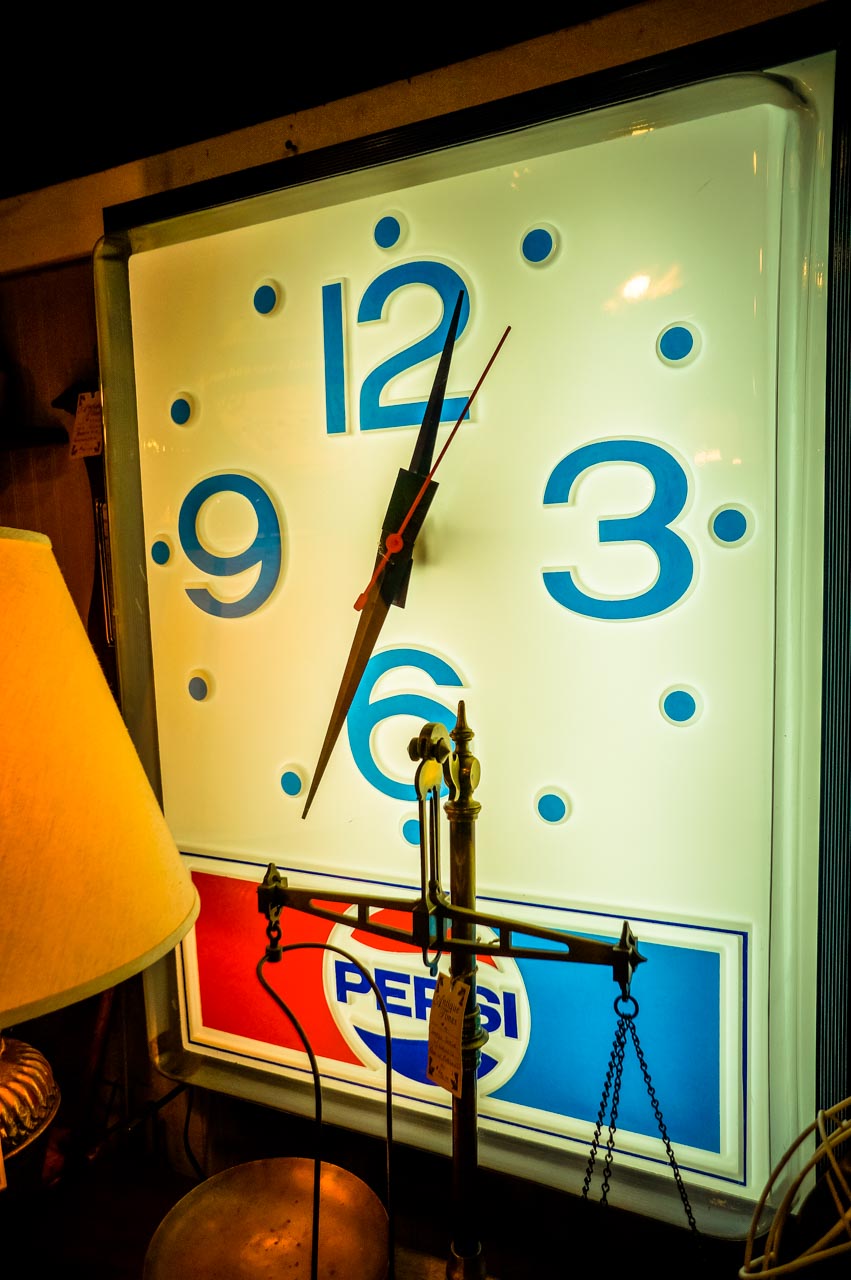In this photo, we see a fascinating collection of vintage knickknacks and relics. Dominating the scene is a striking Pepsi-Cola branded clock, glowing warmly from the illumination inside. The clock, displaying the time 12:34, features a red second hand at the six-second mark and black hour and minute hands. The numbers 12, 3, 6, and 9 are prominent, with simple dots marking the other hours. Flanking the clock on the left is a traditional lamp with a light-colored shade, partially cut off from the frame. To the right, we catch a glimpse of antique balancing scales, characterized by their old-time charm. Though only one scale pan is visible, its distinctive form is unmistakable, adding to the nostalgic ambiance of the scene.